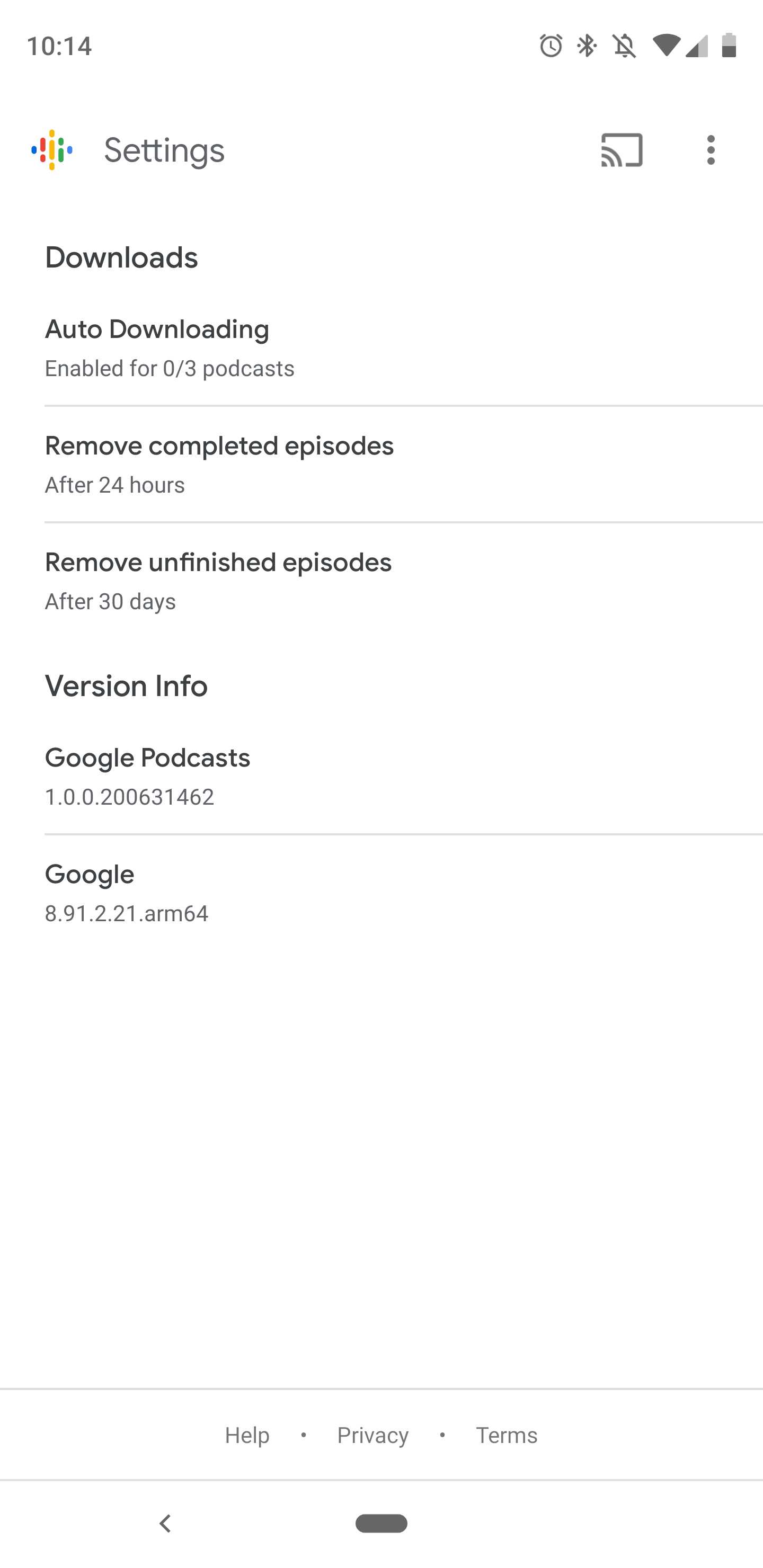This image is a screenshot from a mobile device showcasing the settings section of the Google Podcasts app. The screenshot has a white background and mimics the shape of a long rectangle, similar to a cell phone screen. At the bottom of the screen, two navigation buttons are visible: a back arrow and a silver or gray dash.

The Google Podcasts logo, composed of dots in the Google color scheme (red, green, blue, and yellow) forming a diamond shape, is prominently displayed at the top. Next to the logo, the word "Settings" is written. To the right, there's a Chromecast icon, resembling a TV screen with a Wi-Fi signal in the bottom-left corner, followed by a three-dot menu icon, commonly known as the hamburger menu.

Further down, the screen displays information about downloads: "Auto downloading enabled for 0 out of 3 podcasts" and options to "Remove completed episodes after 24 hours" and "Remove unfinished episodes after 30 days." At the bottom, the version information is listed as "Version info: Google Podcasts" followed by a detailed numerical version number.